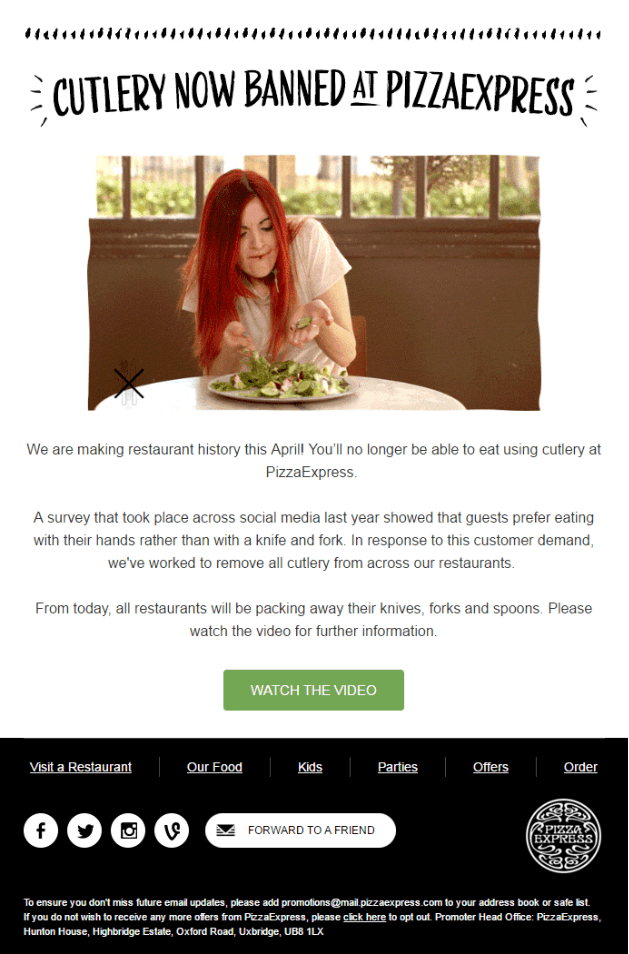The image features a top border composed of various unevenly shaped dots running horizontally from left to right. Below this decorative dotted bar, bold uppercase letters spell out "CUTLERY NOW BANNED AT PIZZA EXPRESS" in large black font, slightly curved at the ends. Positioned beneath this headline is a captivating photograph of a woman with striking red hair, seated at a table set with a plate of food directly in front of her. She appears to be examining a piece of cucumber resting in the open palm of her hand, while her posture is slightly slumped, suggesting a sense of contemplation or disbelief. The caption further elaborates on the scene, asserting that "We are making restaurant history this April. You will no longer be able to eat using cutlery at Pizza Express," thus underlining the significant policy change being depicted.